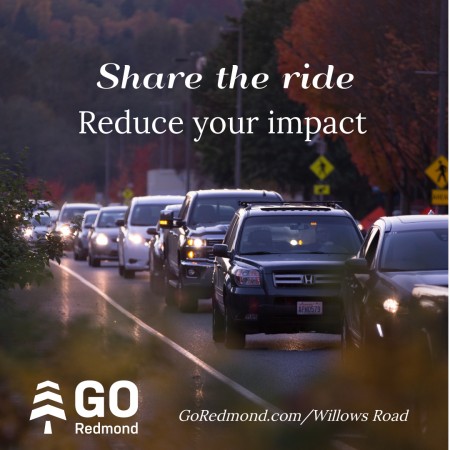In this detailed autumn evening scene, we observe a trafficked road lined with vehicles, predominantly SUVs and sedans, many with their headlights on, suggesting dusk. The image, likely set in Redmond, showcases a mix of red and green foliage against a backdrop of tall trees, potentially hinting at a forest or mountainous area. Prominently, centered at the top in white text, a public service announcement urges, "Share the Ride, Reduce Your Impact," with "Share the Ride" in a distinctive swept font and "Reduce Your Impact" in a more standard, serif typeface. At the bottom left corner, the message "Go Redmond" appears in large, white font, and the bottom right corner directs viewers to "goredmond.com/willowsroad." The overall image maintains a crisp clarity, enhancing the visibility of additional details such as road signs, including a crosswalk sign. This scene effectively combines elements of environmental awareness with the realism of everyday commuter traffic.